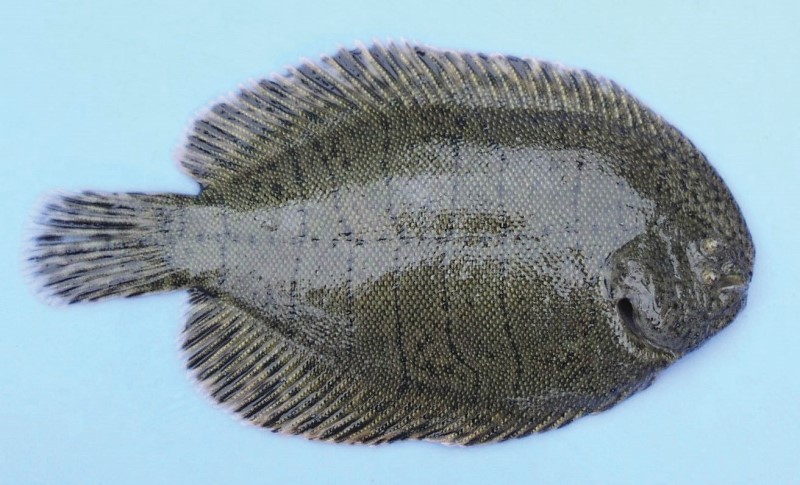This is an image of a deceased, ovular-shaped fish lying on a light blue background, possibly sky blue. The fish has a distinct brownish-tan color with black speckled spots covering its body. Its eyes, unusual in placement, are positioned on the top side of its head, near the mouth, a characteristic of bottom-dwelling fish such as a flounder or rockfish. The fish's body is quite flat, not very three-dimensional, and is designed to blend with the ocean floor, resembling rocks or clumps of sand. It features numerous lines and spines that run vertically from the top to the bottom of its body, with a prominent main line along its spine. Additionally, the fish displays spines on its top, bottom, and tail, which may be venomous, indicated by dark brownish-green and black scales. The gills are located below its eyes, aligned along what can be described as its chin. The fish's camouflage and distinctive physical adaptations suggest it has evolved to thrive in its natural habitat at the ocean or sea bottom.